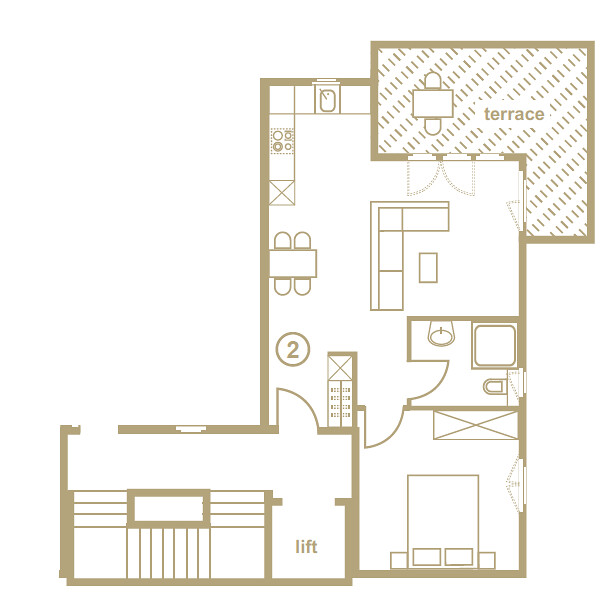This detailed floor plan depicts a beautifully designed single-story house rendered with a white background and elegant gold trim. The layout reveals a well-thought-out space that effectively combines functionality and aesthetics.

Towards the rear of the house, an L-shaped terrace is visible, suggesting a cozy outdoor area for relaxation. Adjacent to the terrace, the kitchen area is distinct, featuring a sink and a stove with four burners, and a dining table surrounded by four chairs, making it a perfect spot for family meals.

The kitchen flows seamlessly into the living room, which is furnished with an L-shaped couch and boasts double doors that open onto the terrace, creating a harmonious indoor-outdoor living experience. Below the living room, there is a bathroom equipped with a corner shower, a sink, and a toilet, ensuring convenience for both residents and guests.

Further to the front of the house, the primary bedroom is located, showcasing a bed flanked by two end tables. To the left of the bedroom, a hallway leads to an area marked as 'lift'. This area features a set of gracefully curving stairs that enhance the architectural intrigue of the home, accommodating upward and downward movement on the left, middle, and right sections of the curved structure.

Overall, this floor plan highlights a harmonious blend of living spaces, promoting both connectivity and privacy within the home.